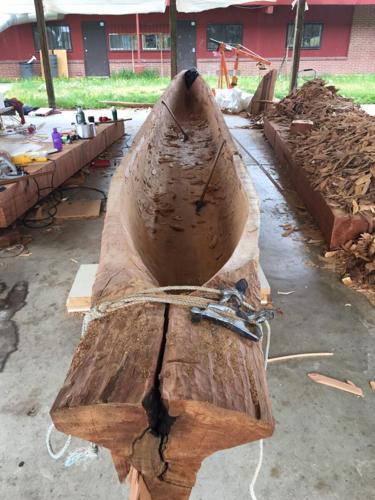In this vertically aligned image taken outdoors during a cloudy day, we see a detailed scene of wood carving in progress under a covered carport. The main focus is a large log being transformed into a canoe. The log, which appears to be a tree trunk, lies on wooden supports and has a large, teardrop-shaped cutout stretching from the bow to the stern. The wood at the back of the canoe has split and is secured with rope. Inside the canoe-in-progress, carving tools and wood shavings are visible.

The carport, with its concrete slab floor, is supported by three wooden posts holding up a white plastic or cloth covering, providing shelter for the workers. On the left side of the image, a wooden table is cluttered with various tools and objects, suggesting ongoing craftsmanship. On the right side, another workbench is covered in wood shavings and bark remnants from the carving process. 

Beyond the open end of the carport, a glimpse of the outdoors reveals a stretch of grass and a building with a red facade, black doors, and several windows. The weather appears to be drizzly and overcast, adding a somber tone to the hardworking scene.